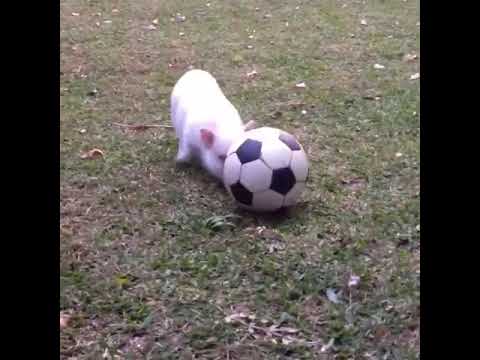In the center of a square photograph, a small, pinkish-white piglet is captured adorably playing with a classic black and white soccer ball. The piglet, characterized by its pink ears and bowing head, is pushing its nose against the soccer ball, seemingly nudging it forward across a grassy field. The grass is a mix of green with brown patches, interspersed with small leaves and flowers. On the ground, a stick lies diagonally from the bottom left to the upper right. The image is bordered by black bars on either side, framing the playful and endearing scene. This quirky photograph emphasizes the piglet's cuteness amidst the natural and slightly untidy grass, bringing a smile to anyone who views it.